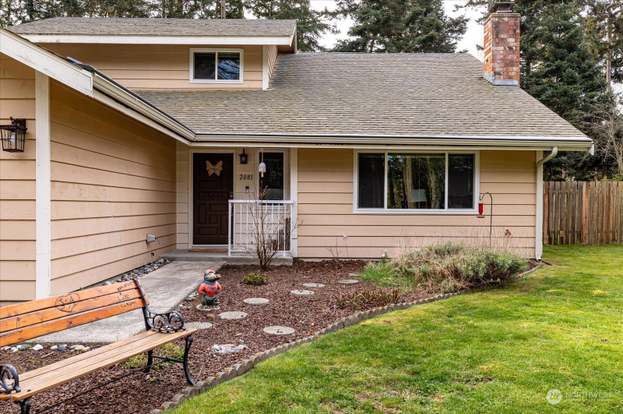This detailed outdoor photograph captures the suburban charm of a two-story, pale brown house with white trim. The front features a dark brown wooden door adorned with a butterfly statue and flanked by a porch light. A single cement step leads up to the door, bordered by a white railing. Nestled to the right of the door, there's a window that adds symmetry to the facade. 

In the foreground, a wooden picnic bench with wrought iron legs and supports rests on a cobblestone pathway that interweaves through a small, somewhat unkempt garden area filled with stepping stones and untrimmed bushes. A small statue graces one of the stepping stones, contributing to the quaint atmosphere. Separating the garden from the lush, green grass yard is a stone border, which extends alongside the walkway.

Behind the yard stands a brown wooden fence, beyond which pine trees and other foliage provide natural privacy. The house itself boasts a gray shingle roof complete with white gutters and a prominent brick chimney. Additional outdoor elements include a classic hummingbird feeder perched on a stand, further enhancing the picturesque suburban scenery.